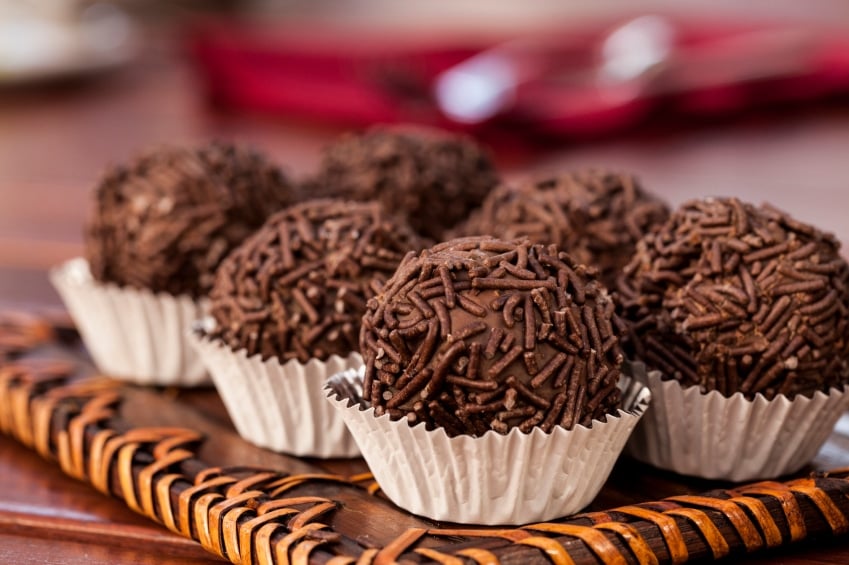This image features a beautifully arranged plate showcasing six chocolate-based desserts. The plate itself has a distinctive design, with a dark brown base color and orange lines decorating the visible left and bottom edges. The interior of the plate maintains the rich, dark brown hue, providing a striking contrast to the desserts. 

Each of the six desserts is ball-shaped and nestled in white cupcake liners. These delectable treats are generously coated with chocolate sprinkles, creating a uniform texture and an enticing visual appeal. 

In the background, the scene becomes blurry, with the table's dark brown color clearly visible in the bottom left corner. This color continues through the image but gradually blurs, transitioning to a gray tone on the right-hand side. Additionally, a blurry red object is noticeable at the top, while a white object can be seen in the top left corner. The very top right of the image fades into a light gray, adding to the overall mystique and focus on the desserts.